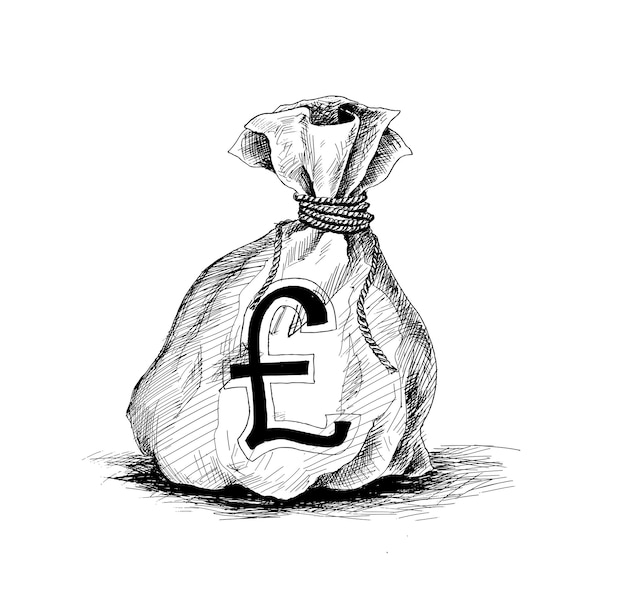This is a black and white pen and ink drawing of a stereotypical money bag, likely made from cloth, tied with a long rope that coils around its neck. The drawing features intricate hatch shading with crisscrossing lines to depict shadows and highlight the bag's lumpy texture. Prominently displayed on the bag's surface, taking up about 70% of the area, is a large British pound sterling symbol (£). The bag appears full and is set against a white background, with dark hatch shading underneath to indicate its shadow. The artwork exhibits decent skill, suggesting it may have been created by a talented high school-aged artist.